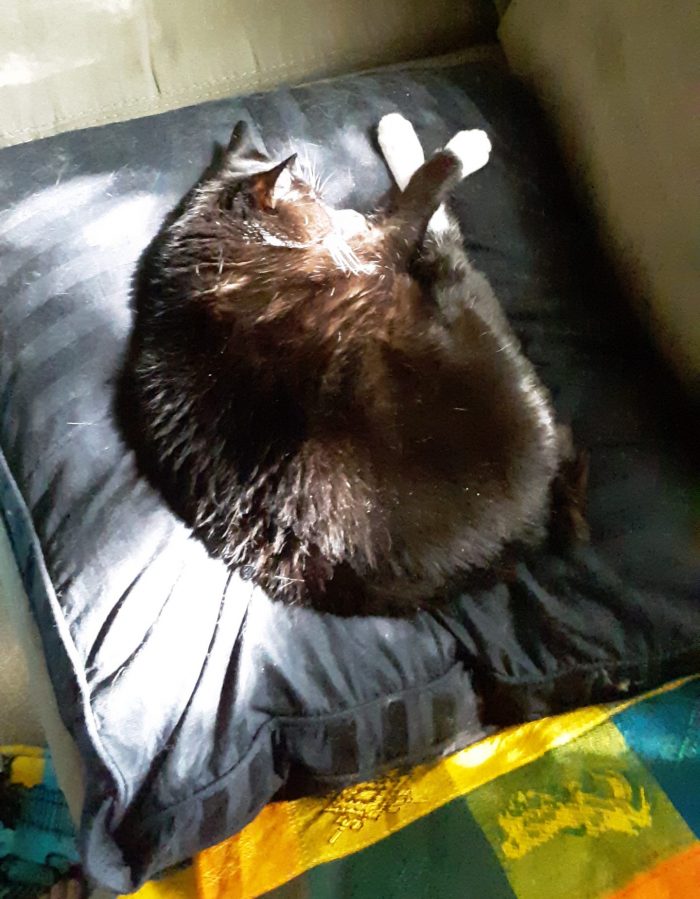A dark brown cat with distinctive white paws is peacefully sleeping in a curled position on a dark gray or black pillow. The cat's right paw is gracefully extended over its bottom rear right paw, which sports a long stripe of white from the ankle to the toes. Its white whiskers are faintly visible as the sunlight filters in, illuminating its face and back, and causing the surrounding fur to glisten. The pillow, adorned with shed cat hair, is positioned on a somewhat dirty beige upholstered couch. Behind the couch and framing the scene is a blanket or pillow in the bottom right corner, showcasing a vibrant criss-cross pattern in yellow, green, blue, and orange. The cat, comfortably basking in the sunlight streaming from an unseen window, appears to be in a serene slumber with its right side facing the camera, which captures the image from an oblique angle, centering the contented feline.